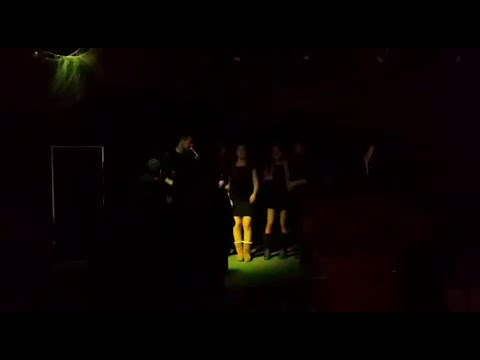This photograph, taken indoors, captures a scene dominated by darkness, punctuated by a faint, greenish light source in the top left corner, likely a spotlight. In the center, partially illuminated by this light, stand four people. On the left, a person seems to be holding a microphone, perhaps singing, though their face is barely visible in the dim light. Beside this person, two women appear to be in dancing poses, their black dresses and legs discernible under the green hue. To the right, another person is mostly obscure, with only their legs faintly illuminated. The green spotlight casts eerie rays, creating a mysterious ambiance. The floor beneath them also reflects a greenish tint. The top and bottom of the image are framed by horizontal black strips, intensifying the overall darkness.